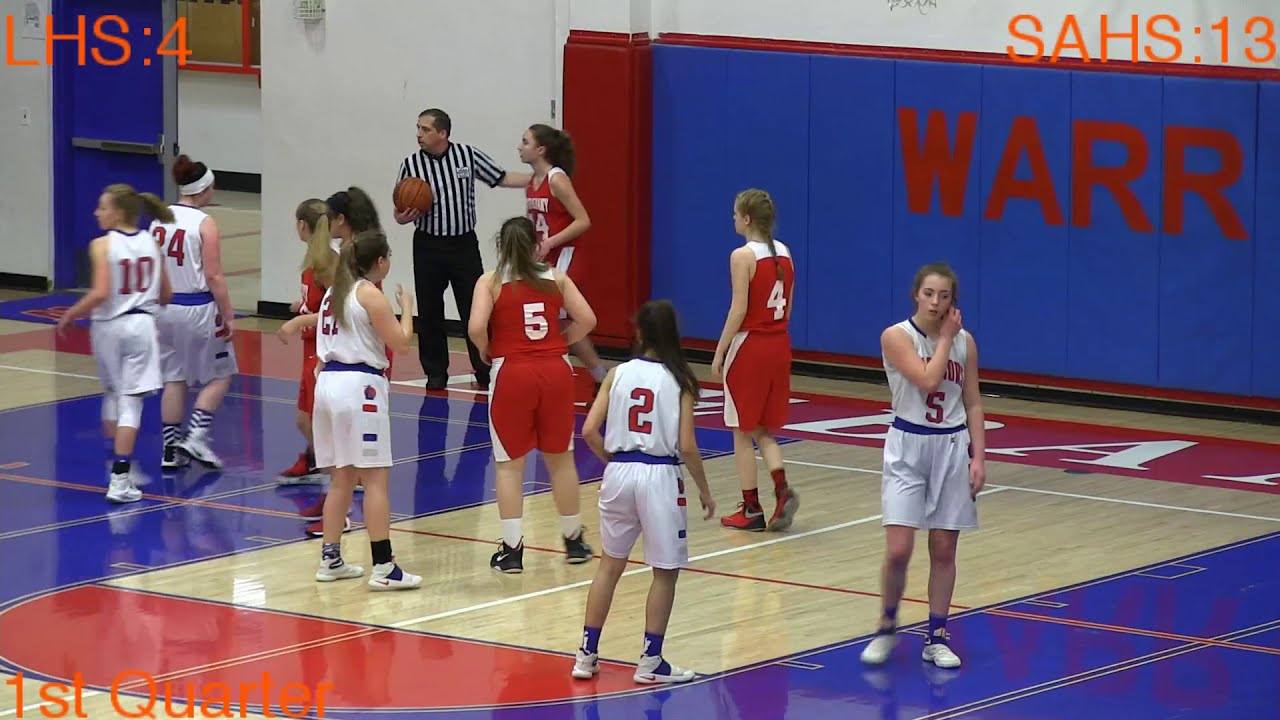The photograph, taken indoors in a high school gymnasium, captures a moment from a girls' basketball game. The glossy wood grain floors, marked with typical basketball court lines, set the stage. The image features players from two high school teams: one team in white uniforms accented with red and blue, and the other in red uniforms with white accents. The referee, holding the basketball and preparing to resume play, stands at the center of the scene with his arm extended toward a player in red, possibly indicating an inbound pass. The players appear to be in position, with the white team ready to defend. The text overlay on the image provides details about the game: in the upper left corner, "LHS 4" in orange; in the upper right corner, "SAHS 13"; and in the lower left corner, "First Quarter." The background reveals a white wall with blue padding and part of the home team's name, "WARR," in red, likely short for "Warriors." The overall score and the game context suggest it is the first quarter, with SAHS currently leading.